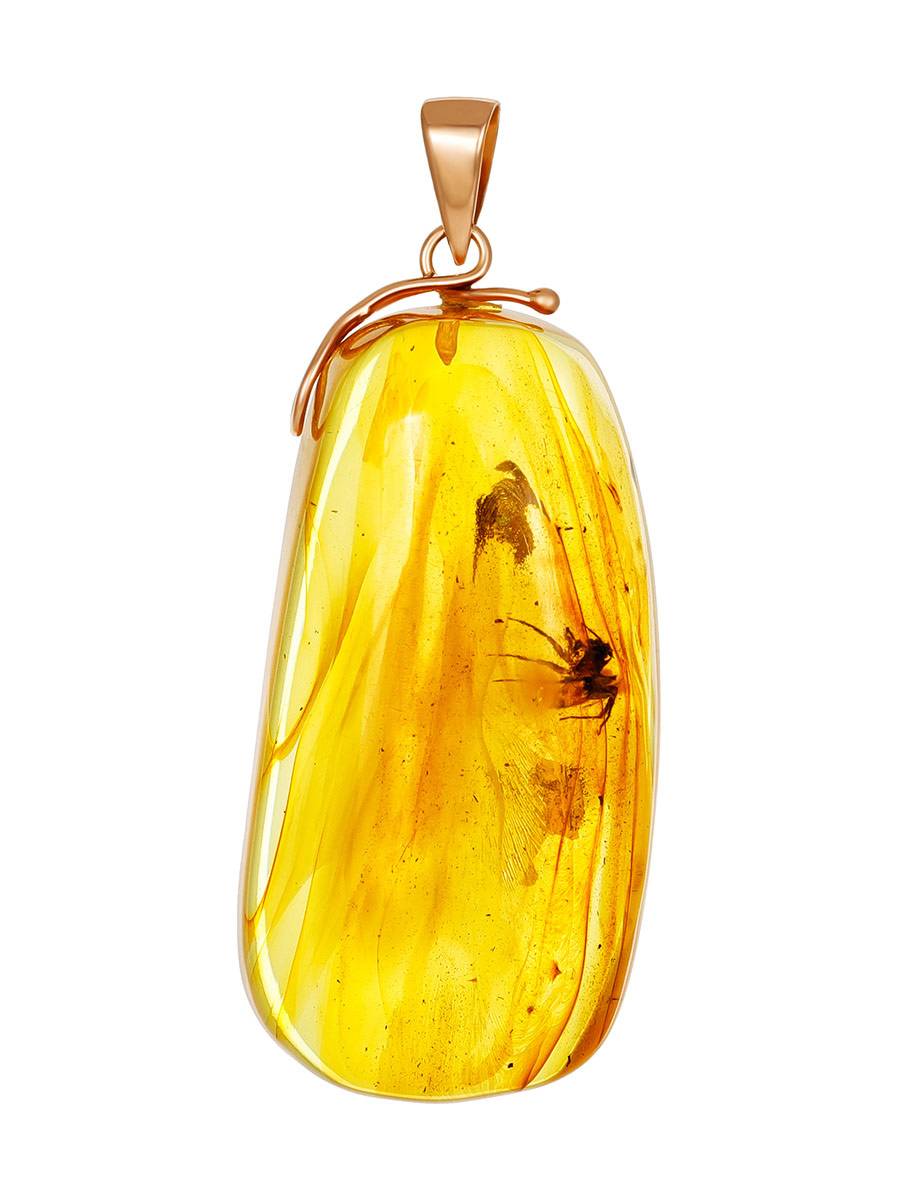The image showcases a shiny, golden-yellow pendant that appears to be a standalone charm, not yet attached to a necklace. This oblong, oval-shaped pendant features intricate gold fittings at the top, including a hoop and a clasp. The stone itself is primarily yellow, embellished with flecks of tan and brown that create a unique pattern. Some darker brown streaks within the yellow give an impression of a spider or insect, though it's merely a visual effect of the stone's natural inclusions. The pendant, boasting a smooth and rounded form, is set against a plain white background, devoid of any text or additional elements.